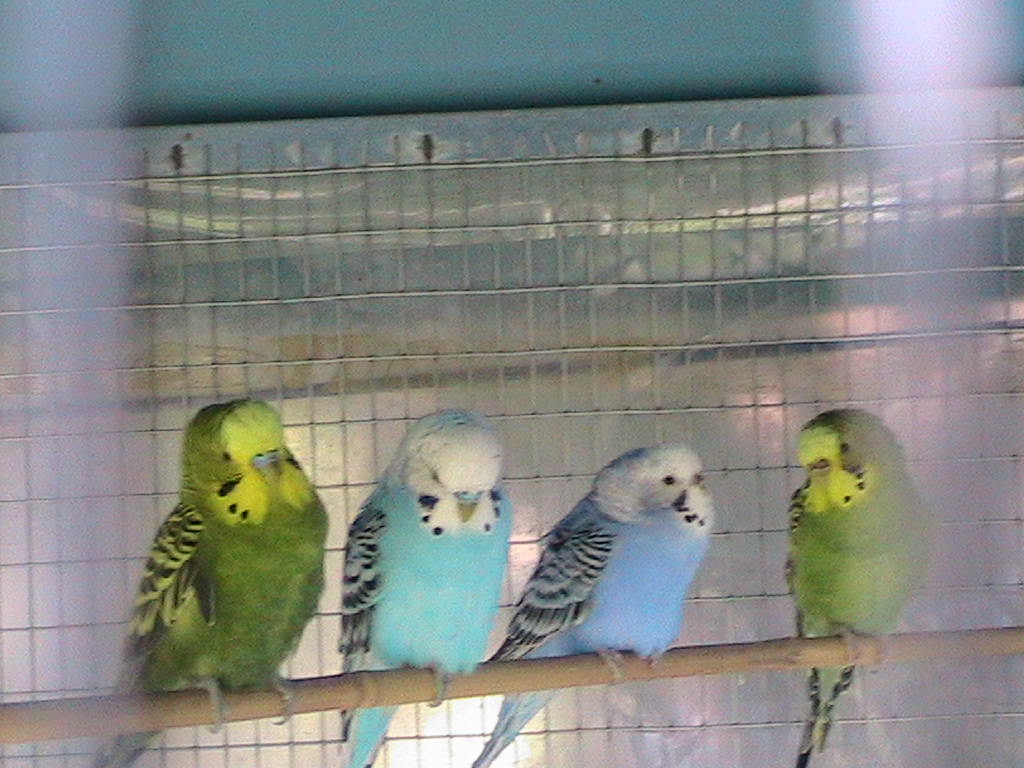The image captures four parakeets, each perched on a light brown twig that stretches horizontally across the interior of a metal cage with silverish bars. The foreground includes blurry metal bars indicative of the picture being taken through the cage. The leftmost and rightmost parakeets are nearly identical, both displaying a vibrant green body with a yellowish face and black markings on their wings. The two middle parakeets differ slightly in color. The second bird from the left boasts a pale blue body with a white face and black and white wings. Next to it, the third bird showcases a deeper blue or purplish belly, also accompanied by a white face marked with some gray and distinct black and white wings. The scene captures the vibrant, tropical allure of these colorful parakeets in their enclosed habitat.